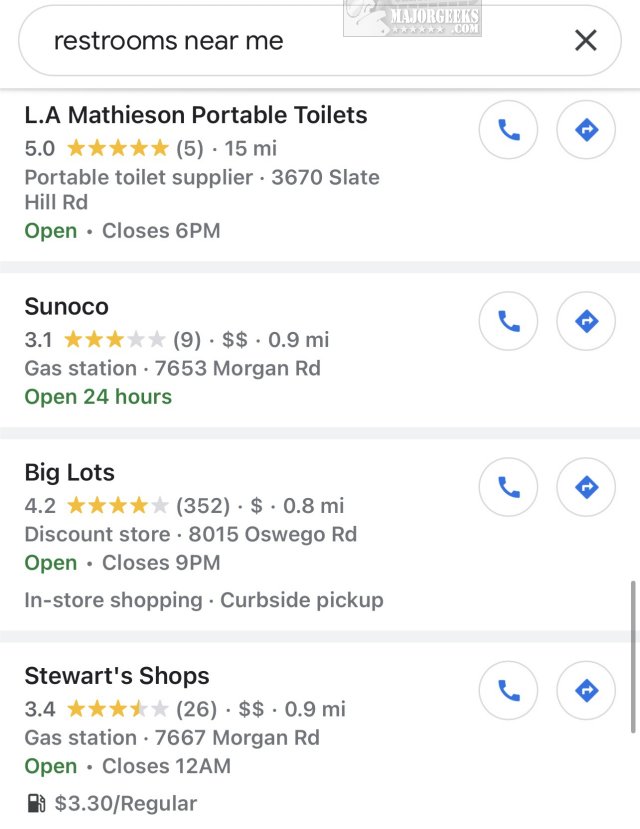The image displays the results of a Google search for "restrooms near me." Four establishments with restroom facilities are listed, complete with ratings, distances, types of establishments, hours of operation, and additional features. 

1. **L.A. Matheson Portable Toilets**: Rated 5.0 stars, this portable toilet supplier is 15 minutes away. Located on State Hill Road, it is currently open and will close at 6 p.m.
 
2. **Sunoco**: A gas station with a 3.1-star rating, it operates 24 hours a day.

3. **Big Lots**: This discount store holds a 4.2-star rating and is 0.8 miles away. It is open and will close at 9 p.m.

4. **Stewart's Shops**: With a 3.4-star rating, it is 0.9 miles away. This shop is open and will close at 12 a.m.

Each listing includes clickable phone icons and direction buttons, both highlighted in blue, providing users with convenient ways to contact or navigate to these locations.